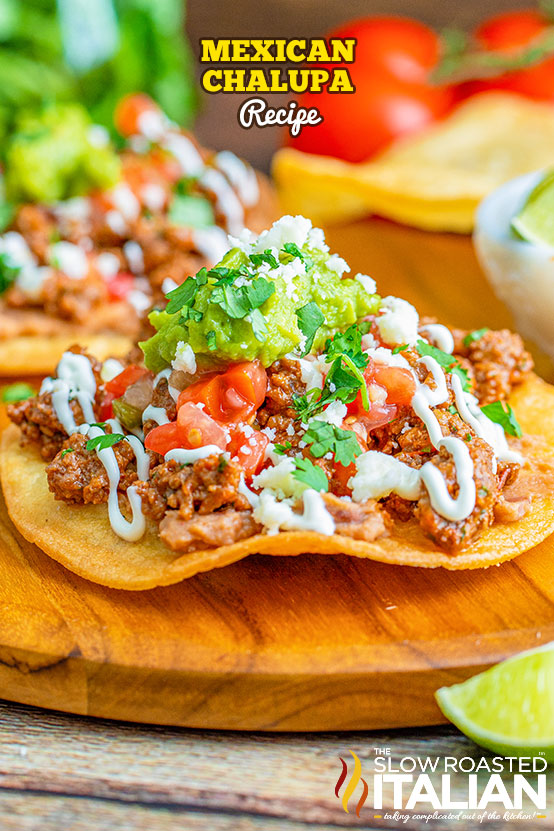This indoor photograph prominently features a vivid display of a Mexican chalupa recipe. At the top, bold yellow letters with a black outline spell out "Mexican Chalupa," while the word "recipe" appears in cursive white writing, also outlined in black. Centered in the image is a wooden cutting board holding an open tortilla lavishly topped with salted ground beef, creamy guacamole, cilantro, crema, diced tomatoes, beans, onions, and a drizzle of a savory sauce. Off to the side, partially visible, is a slice of lime, suggesting a serving accompaniment. The blurred background artfully showcases additional tortillas, a vine of fresh tomatoes, and another out-of-focus chalupa, enhancing the scene with an authentic kitchen atmosphere. Situated on a wooden table, the scene is complemented in the bottom right corner by a logo featuring yellow and red flames, with white letters spelling out "The Slow Roasted Italian," indicating the likely source of this tempting recipe.